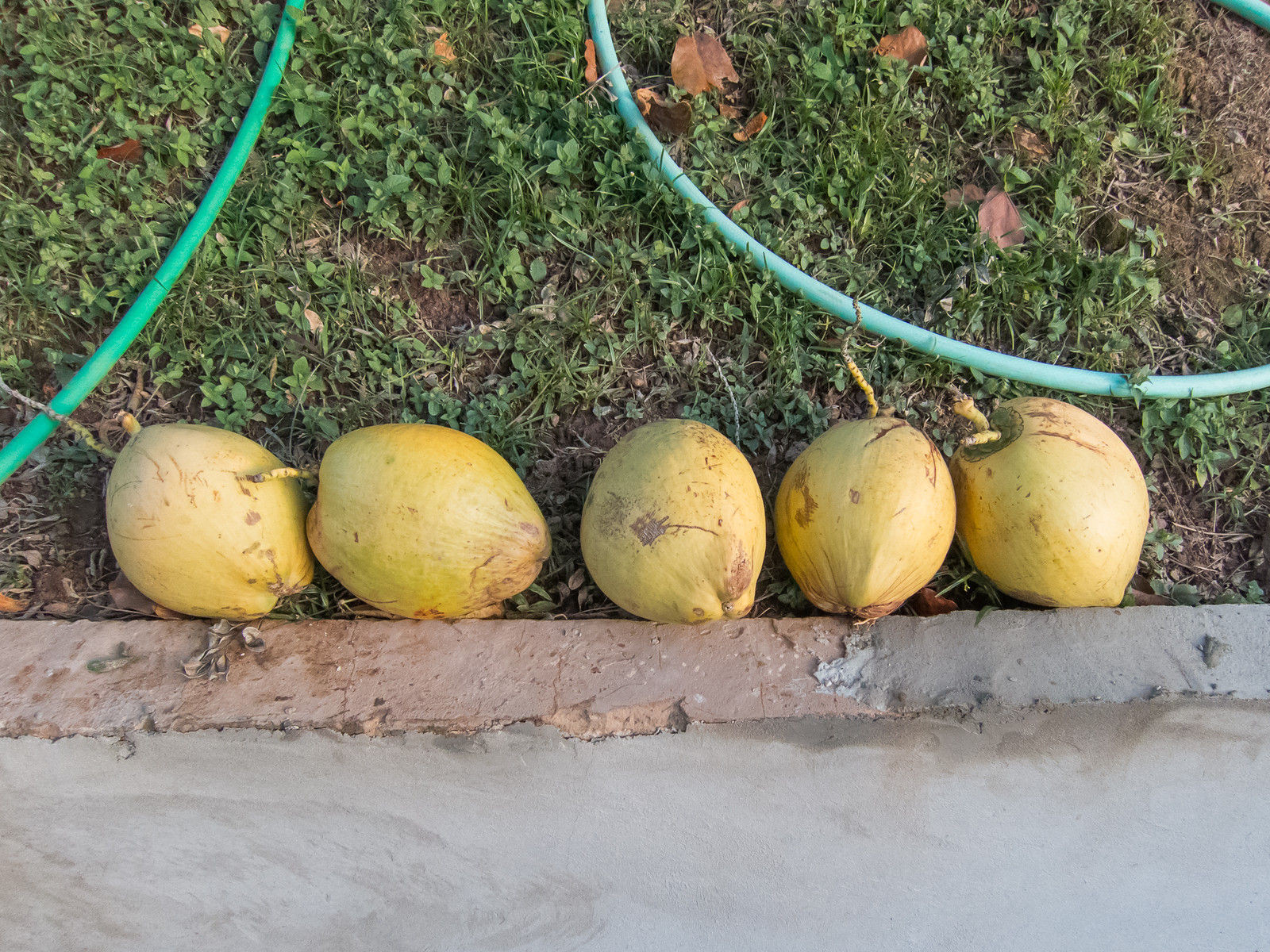The image captures a line of five yellowish, slightly oblong fruits resting on a gray cement ground bordered by a red and gray brick paver before transitioning into an area of grass and dirt. The fruits, possibly figs or small gourds, are arranged in different orientations — some leaning left, some right, and one facing forward. Each fruit has a yellow skin with brown patches and a couple feature small stems. Above the fruits, a green garden hose snakes through the grass, appearing in the upper left and upper right corners of the photograph. The grassy background is interspersed with a few brown leaves, adding a touch of the natural outdoor setting.